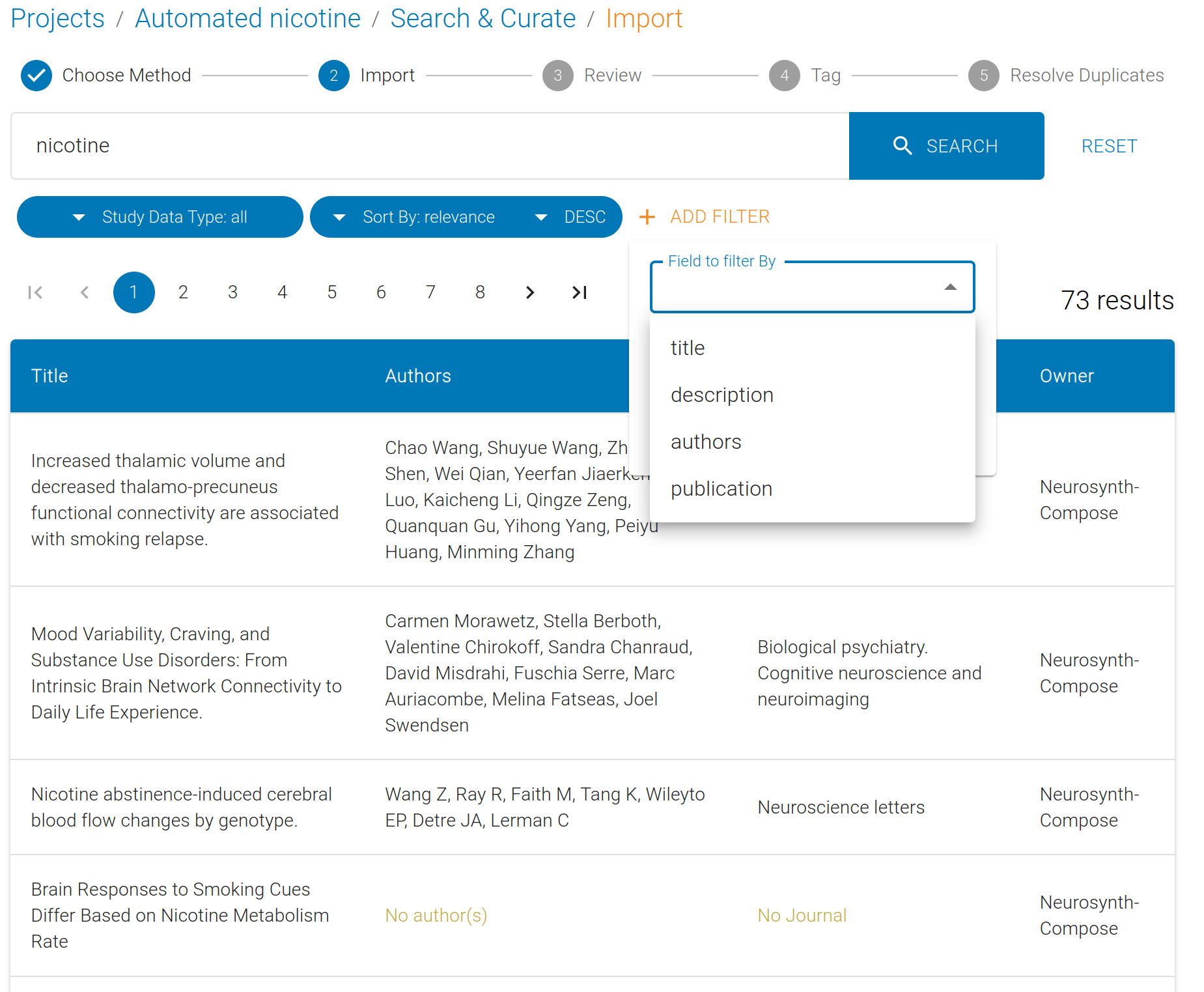The top left section of the interface displays the following tabs: "Projects," "Automated Nicotine," "Search and Query," "Import." Below these tabs, a blue checkmark indicates the selected method for the import process. The steps outlined are:

1. Choose Method
2. Review
3. Add Tag
4. Resolve Duplicates

There is a blue rectangle marked "Search" with a "Resend" option, followed by a field for inputting data less than nicotine.

A blue triangle highlights "Study Data Type," set to "All," indicating relevance. There is an option to add filters based on title or description for the publication, displayed on the right side of the interface with results shown on the left.

A red arrow points to a sequence, marked by blue circles numbered one through nine. Another red arrow, specified by a left vertical line, is also present. The row under the blue rectangle categorizes data into "Title" on the left and "Authors" on the right. 

The first title listed is: "Increase in Labic Volume and Decrease in Precutaneous Functional Connectivity Are Associated with Smoking Relapse," by authors Chao Wang, Shuyi Wang, Shen Wei, Qian Yifan, Jie Luo, Kai Sheng Li, Xinxin Zeng, Guangkuan Gu, Yihong Yang, Aiyu Yuan, Huang Mingming, and Zong Mingming. This publication is indicated as coming from Neurosynth.

The second title is: "Mood Variability, Craving, and Substance Use Disorders from Intrinsic Brain Network Connectivity of Daily Life Experience." 

Another title listed is: "Nicotine Abstinence Induced Cerebral Flow Changes by Genotype."
 
The final listed title is: "Brain Responses to Smoking Cues Related to Nicotine Metabolism Rate."